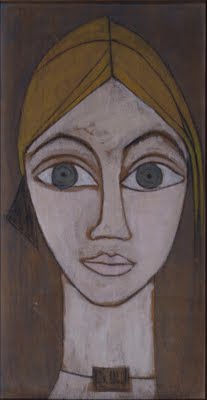The image is a painting of a woman's face executed in a highly stylized and creative manner. The focal point is her face and elongated neck, positioned centrally on a vertically-oriented canvas. She has exceptionally large eyes, thin eyebrows, full lips, and a long nose. Her hair, which could also be interpreted as a cap, is blonde. The woman's neck extends unnaturally long, reaching the bottom of the painting, without showing her body. She wears a necklace or piece of jewelry around her neck. The background is predominantly dark brown, complemented by various colors including light brown, tan, blue, white, gray, and green, accentuating the light pink tone of her skin and the grayish hue of her eyes. The overall style is abstract and the painting could be typically seen in an art show, with no text or additional objects present in the image.